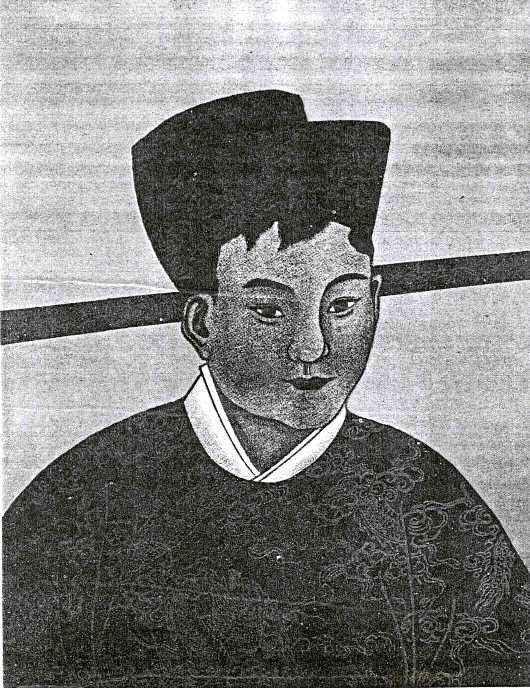This detailed black-and-white sketch portrays a young Asian man with dark black hair partially obscured by a black hat, from which his bangs emerge. Uniquely characterized by elongated, slightly slanted eyes, the man wears what appears to be a traditional Japanese kimono adorned with an ornate pattern, suggestive of common historical designs, such as dragons. The kimono is complemented by a white collared shirt beneath it and details intricate frills. The background features a textured, dual-tone gray setting with a horizontal black rod across the middle section behind the man’s head, creating a stark and artistic contrast. The entire image is rendered in a meticulous, grayscale artist's rendition, capturing both cultural attire and personal expression without any accompanying text.